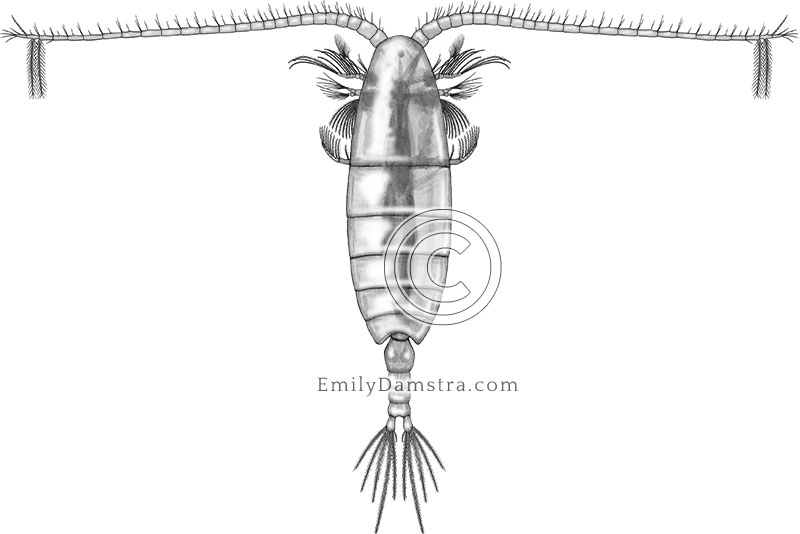This highly detailed, monochrome drawing by Emily Damstra depicts a peculiar and possibly deep-sea creature, characterized by its intricate features. The creature has a translucent, segmented, oval-shaped body adorned with fine striations, devoid of visible legs or arms. Extending from its head are long, fuzzy antennas, each spreading outward to the sides like a drafting T-square, adding to its eerie yet delicate appearance. The central section of the body showcases various hair-like cilia protruding from multiple areas, enhancing its otherworldly look. At the bottom, there's a small, ambiguous appendage that could be a tail or a pincher. The entire composition is presented against a stark white background, emphasizing the creature's ethereal and obscure nature. The drawing includes a copyright symbol and the artist’s signature web address, emilydamstra.com, confirming the artwork's authenticity and creator.